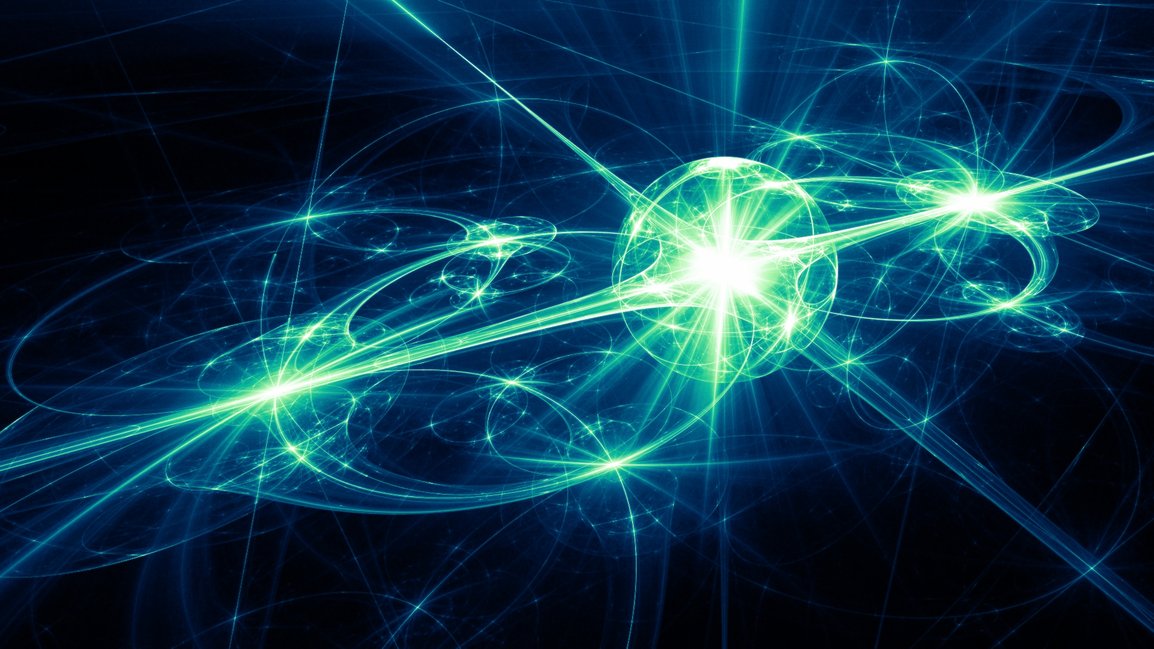This computer-generated artwork features a dark blue and black smoky background, giving it a mysterious and sci-fi ambience. The design is centered around a large, bright green orb positioned slightly off-center to the right, from which vivid beams of white light radiate in four directions. These beams connect to smaller, less vibrant orbs, creating an intricate web of interconnected energy points. Swirls, light marks, and delicate lines of mint green energy flow across the image, contributing to its dynamic and magical feel. The sides are not perfectly symmetrical, with various subtle light points scattered throughout, enhancing the sense of an outer space or cosmic energy flow. The scene is both bold and mesmerizing, capturing the essence of an otherworldly energy field.